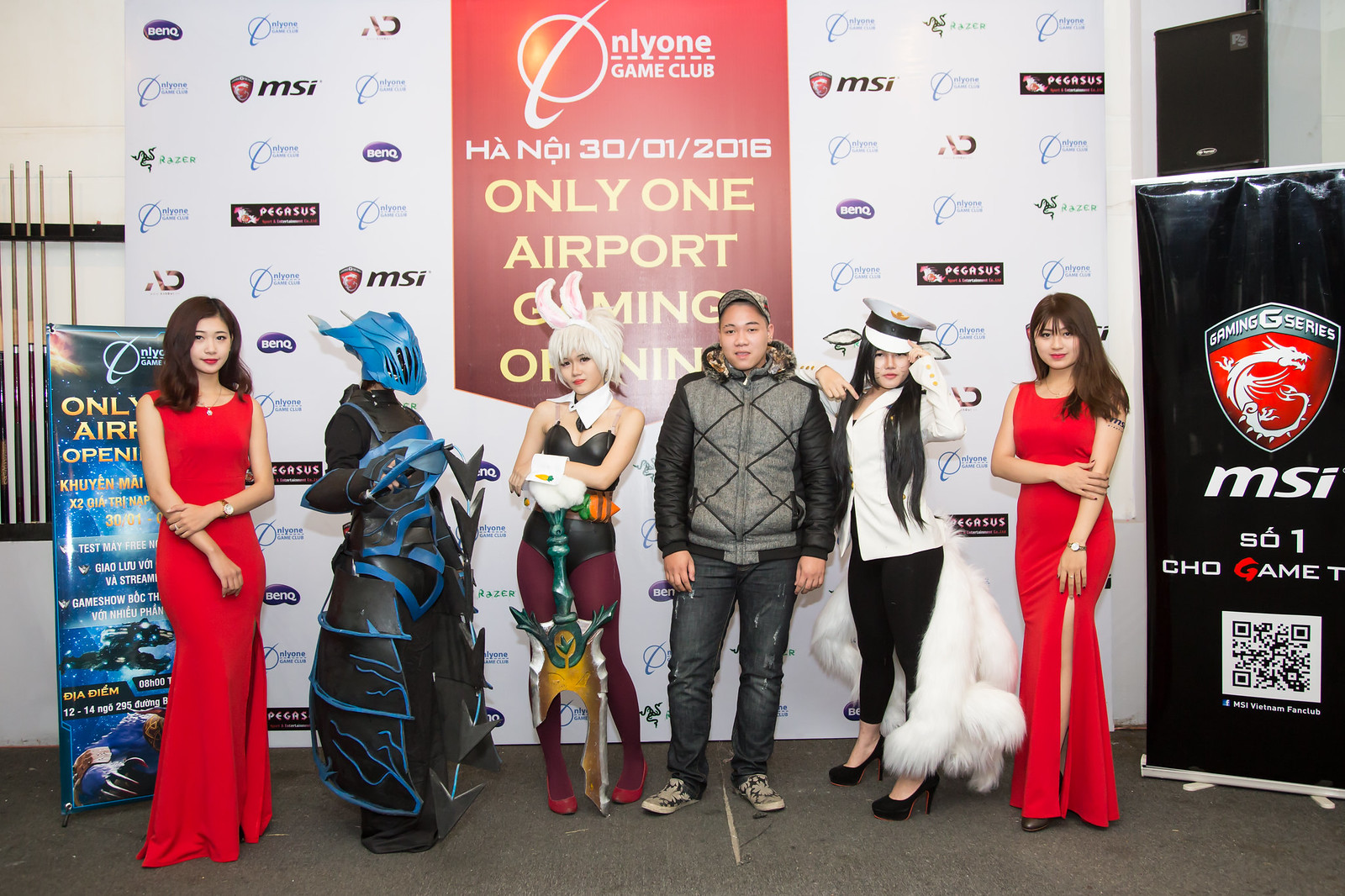The photograph, taken indoors, captures six people standing in front of a board that reads "Only One Airport Gaming" and "Only One Game Club." This suggests the event is gaming-related and possibly held in Vietnam, as indicated by the text "Hanoi 30 Jan 2016" on the banner. Among the six individuals, four are in the center and dressed in elaborate costumes, suggesting a cosplay event.

On the leftmost side, two Asian ladies, presumably models, wear long, red sleeveless dresses. Each has one arm bent at the elbow, crossing their stomach and holding the other arm. Next to them, a person is fully clad in a black costume with a blue, full-cover mask and helmet, hiding their face completely. 

In the center stands an Asian man dressed in plain clothes, indicating he is not partaking in the cosplay. To his right, an Asian lady adorned with bunny ears wields a large green and gold sword, while another Asian lady, standing with her arm on the plain-clothed man's shoulder, sports a sailor hat, a white dress coat, and black pants. She features drawn whiskers on her face and has nine white bushy tails, completing her cosplay outfit.

All individuals appear to be on a stage, possibly at a convention hall, marked by a backdrop mentioning "Only One Airport Gaming Online." The attendees and those in the photo predominantly look Asian, aligning with the event’s likely setting in Vietnam.